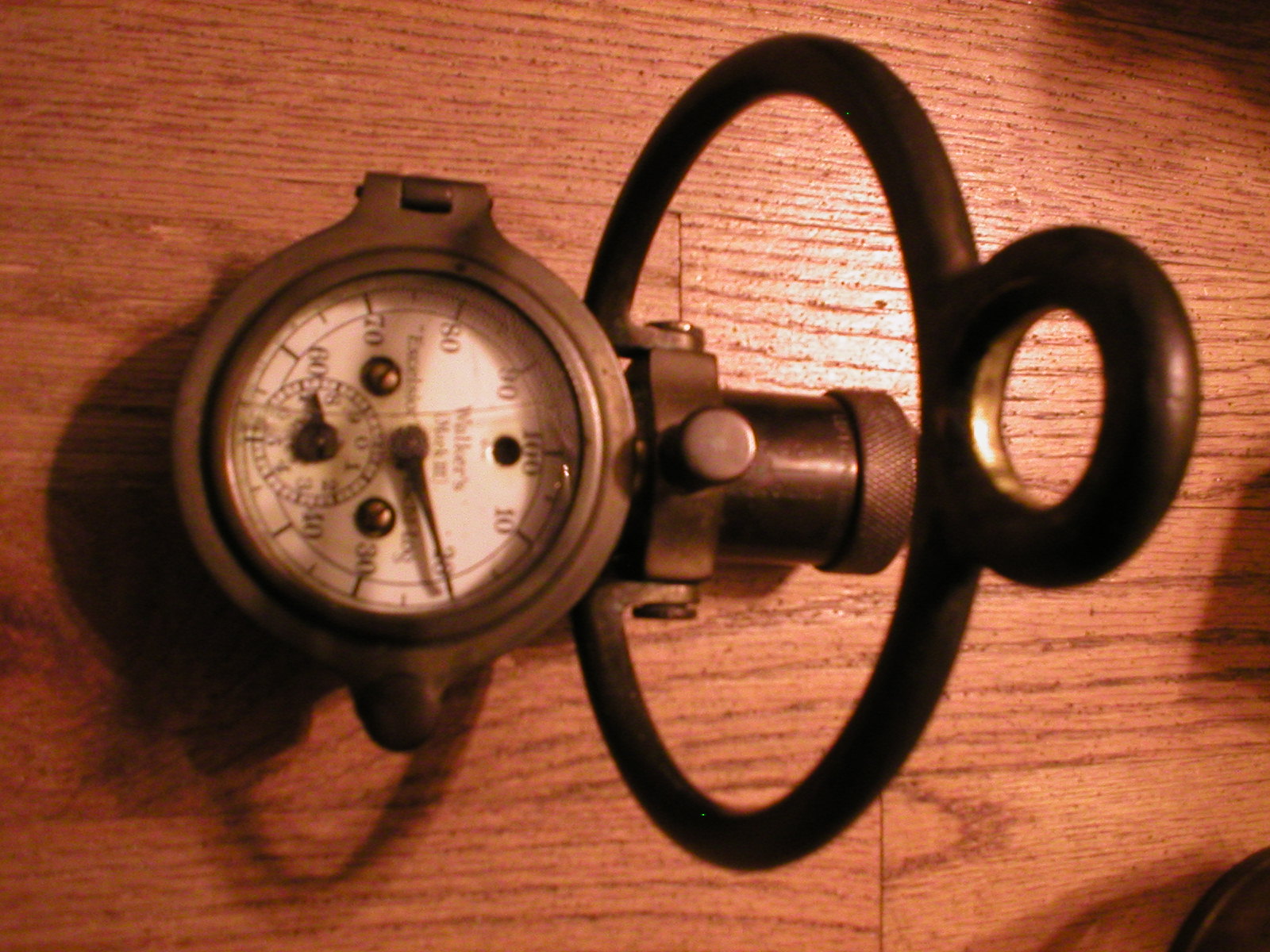The image showcases a detailed close-up of a horizontally placed pressure meter. The background consists of a light brown wooden texture, likely a wall or a table. The meter is positioned such that you need to turn your head to the right to read it properly. The meter features a white face with brown numerals, starting from 100 at the top and decreasing by increments of 10 to 50 at the bottom. Conversely, the numbers 60, 70, 80, and 90 are outlined with dashed lines, moving from the center towards the left. A dark brown handle, set at the 20 mark, serves as the dial. The outer rim of the meter is also brown, complementing the overall color scheme.

To the right of the meter, a brown loop is visible, accompanied by a smaller, similarly colored loop above it. Additionally, there is a gray knob capped by another knob-like structure at the end of the object. Shadows are cast in the top right and bottom right corners, accentuating the wooden table that forms the entire background of the image.